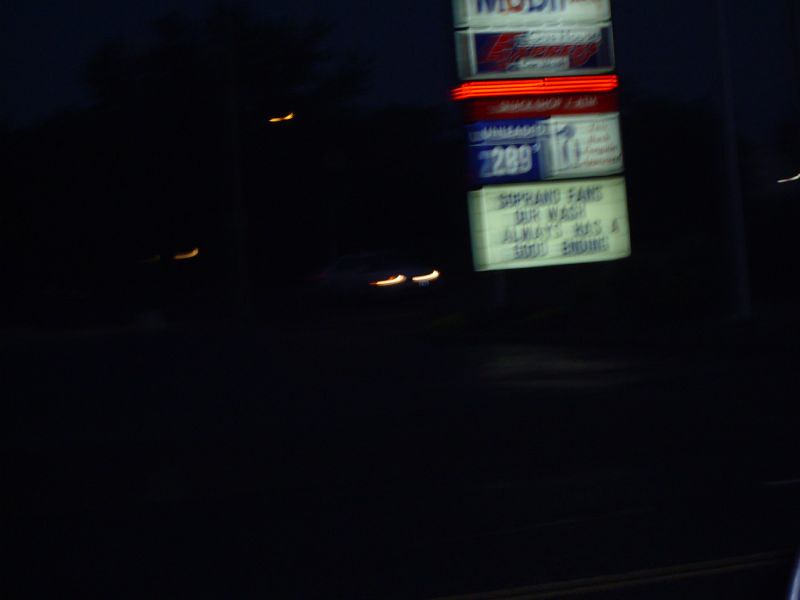The image, taken at night, depicts a dimly-lit exterior scene dominated by a gas station sign in the upper right corner. The sign, presumably belonging to a Mobil gas station, features blue and red writing with the incomplete logo "MOB". Below this, a red band divides the sign from a digital display indicating the price of unleaded gasoline at $2.89 per gallon. Adjacent to the price is an advertisement featuring a penguin facing left, though the accompanying text is unreadable. To the left of the gas station sign, the image reveals faint car headlights, suggesting nearby activity. Additional signage includes a blurred reader board with black letters on a white background, partially decipherable with phrases like "Soprano fans" and "our wash always". The overall scene is characterized by its darkness, with only a few scattered lights providing minimal illumination.